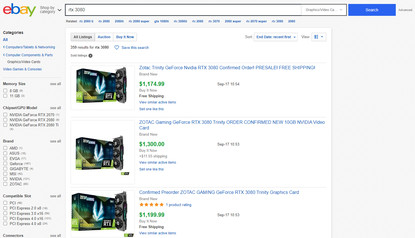The screenshot captures a search results page on eBay, specifically focused on computer equipment, likely a graphics card, although the image details are blurred. Dominating the upper left-hand corner is the iconic eBay logo, with each letter in a distinct color: E in red, B in blue, A in yellow, and Y in green. Adjacent to the logo is the search bar where the query was entered, followed by a blue search button.

Directly below this are various subheadings that appear to offer further options to refine the search results. To the left side of the screen, a vertical column lists categories and filters, enabling users to narrow their search by selecting more specific criteria.

On the right side of the screen, the actual search results are displayed. Each item is presented with a thumbnail image, individual pricing, and a link to its product page, which is denoted in blue text. The background for the listed items is white, while the surrounding border area is light gray, providing a modest visual contrast between the individual listings and the overall page layout.